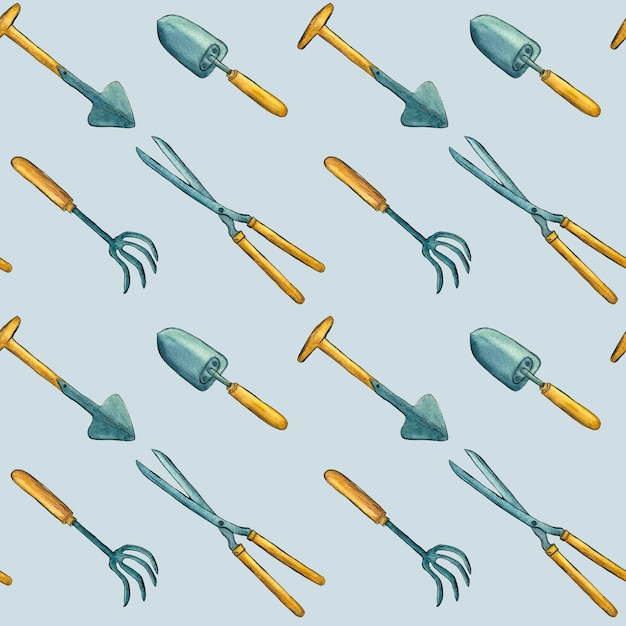This image appears to be a hand-painted pattern, reminiscent of wallpaper, set against a pale, light baby blue backdrop. The central theme revolves around garden tools depicted in a repeating series. These tools, each with golden or brown handles, likely wooden, and darker blue-gray metal tops, include an assortment of shovels, spades, handheld rakes, hedge trimmers, claw weeding tools, and shears. The arrangement follows a specific sequence: starting with a small hand shovel, followed by a garden spade, a claw weeding tool, and shears, creating a diagonal alignment. The detailed depiction emphasizes the universal nature of these gardening tools, arranged meticulously to create a uniform, repetitive pattern.